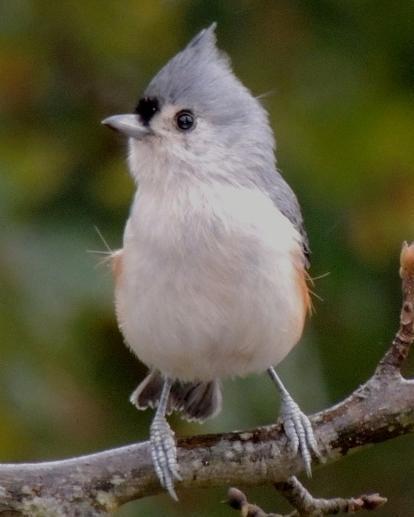This captivating close-up photograph features a small bird perched on a slender, twig-like branch, set against a beautifully blurred outdoor background filled with hints of green foliage, suggesting a natural setting such as a forest or neighborhood garden. The bird, possibly a chickadee, is characterized by its striking color palette: it boasts a predominantly gray plumage with a slightly pointy head, accented by a distinctive black spot just above its gray beak. Its underbelly and the lower part of its head are a contrasting creamy white. Subtle splashes of orange or brown are discernible on either side of its body, near the wings, adding a touch of warmth to its otherwise cool-toned feathers. The bird's black, beady eyes give it a charmingly alert expression. Its scaly gray feet grasp firmly onto the brown branch, grounding this delicate avian in its natural environment.